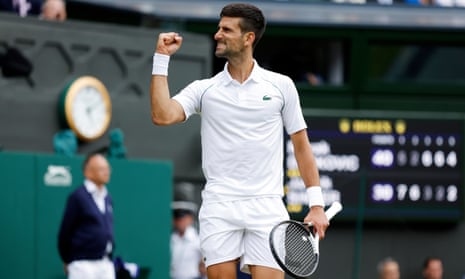This vivid color photograph captures a triumphant tennis player centered in the frame. The player's attire is all white, consisting of a short-sleeved shirt, shorts, and wristbands on both arms. His right fist is raised in celebration while his left hand holds a tennis racket. The player is dark-skinned with dark brown hair and light facial hair. Behind him, the blurred background reveals details of a tennis court, including a green wall, a clock, and a digital scoreboard. To the left, there is an indistinct figure that appears to be a man wearing a navy hat, navy sweater, white shirt, and white pants. The image encapsulates a moment of victory and the ambiance of a tennis match environment.